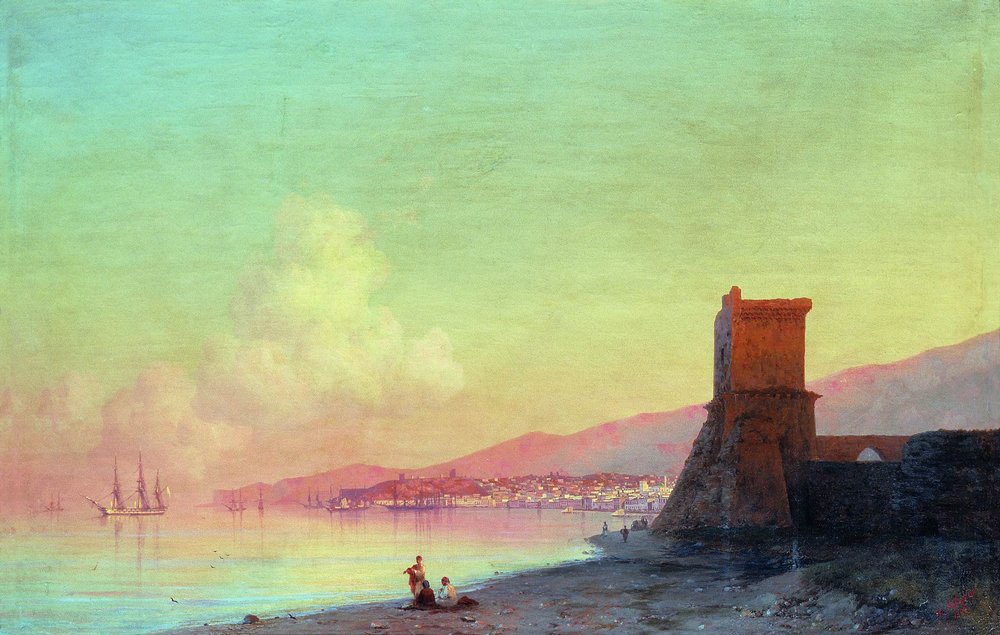This outdoor painting captures a breathtaking scene at what appears to be dusk or dawn. The sky gracefully transitions from teal and blue at the top, shading down into vibrant pink and yellow hues near the horizon. A bank of fluffy white clouds occupies the sky's left side above a calm, light blue body of water that reflects the serene sky. The water is home to several ships with cloth sails and masts, the most prominent being an old-style sailing ship with three masts.

On the left-hand side of the image, the rocky beach meets the tranquil water. Three people are seated on blankets in the foreground, facing the bay—two sitting while one stands. The beach appears a mix of sand and scattered rocks, with a few more figures strolling in the distance toward the right.

Towards the right side of the picture stands a tall stone structure resembling a tower or observation point. Attached to this structure are stone walls extending off the image’s edge. Behind these walls, a village or town with numerous buildings nestles at the foot of a towering mountain range, which spans from the middle right to the left-hand side in the background, creating a natural boundary for the bay. The intricate details of the landscape, combined with the soft pastel tones of the sky and water, evoke a sense of tranquil beauty and timelessness.